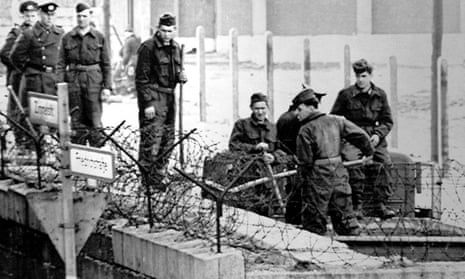This vintage black-and-white photograph captures a wartime scene featuring multiple soldiers in military attire standing behind a barbed wire fence. In the foreground, a stone wall topped with barbed wire encloses the area, and a post with two unreadable signs points in opposite directions. Towards the back, slightly out of focus, a row of wooden fence posts and a distant brick-walled building can be seen. On the left, three soldiers stand in a row, with one wearing a commander's hat and the others donning lower-ranking uniforms; they stare forward with a look of vigilance. Nearby, another soldier stands alone, peering over the barbed wire with a strained expression. To the right, a soldier stands with a shovel, watched by two seated comrades. Additionally, several soldiers on the right appear to be carrying a large black object or shoveling items from a rectangular box. The image captures a mix of stationary and active soldiers, reflecting a tense and busy wartime environment.